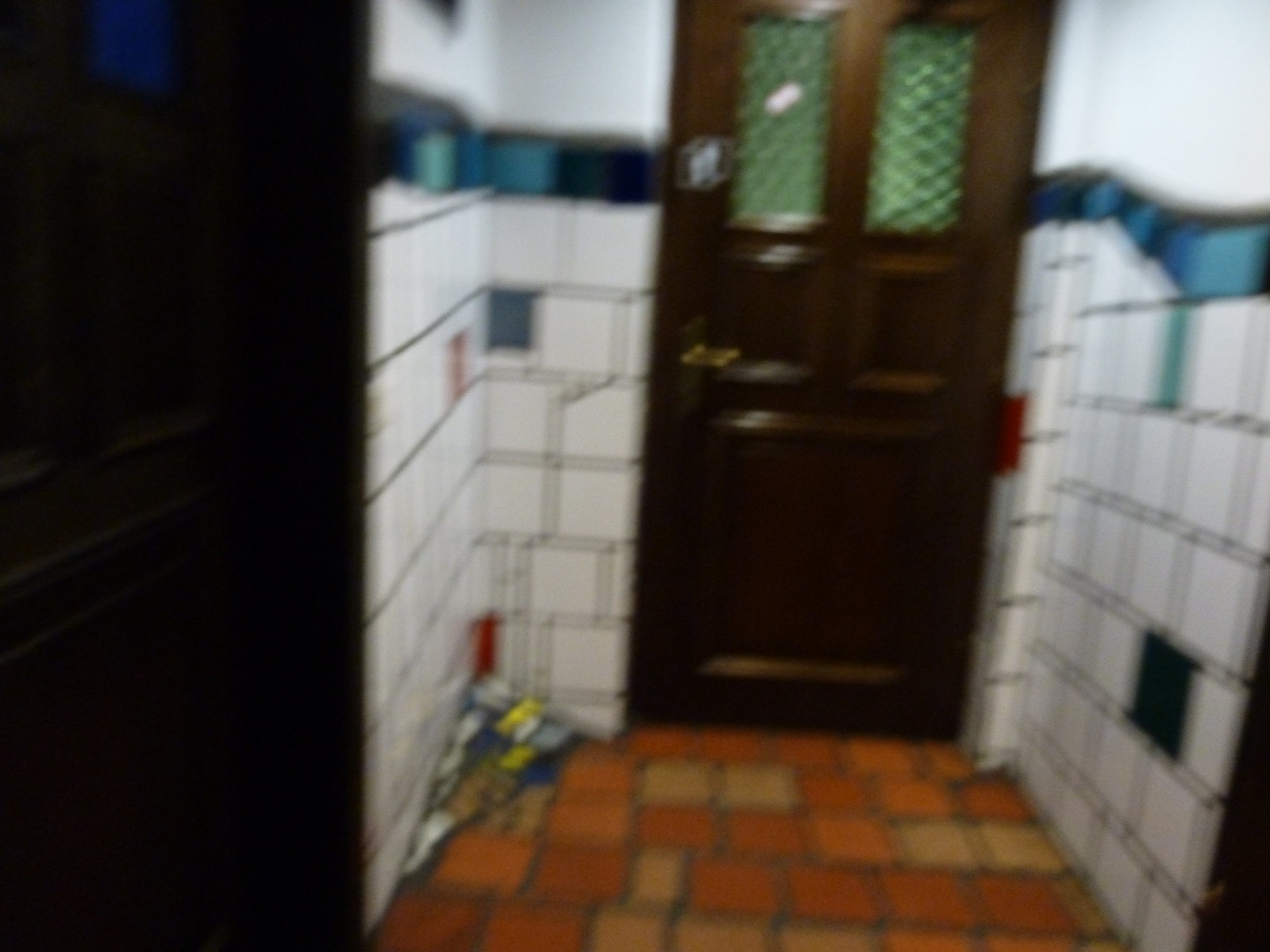In this blurry photographic image, a long wooden door with two side-by-side windows, framed by panels, stands prominently at the end of a hallway or foyer. The glass panes in the door feature distinctive green and black lines. The left side of the image shows a black area, while the upper portions of the left and right walls are white. The bottom half of the walls is adorned with mostly white tiles interspersed with various shades of blue and occasional red tiles, creating an artistic and diverse pattern. The tiles vary in shape, including squares and rectangles, contributing to the dynamic visual composition. The floor is covered in square tiles of varying hues, including dark orange, burnt orange, yellow, and brown. A noticeable object, possibly a triangular school banner, is located in the left-hand corner of the floor, adding an element of intrigue to the scene.